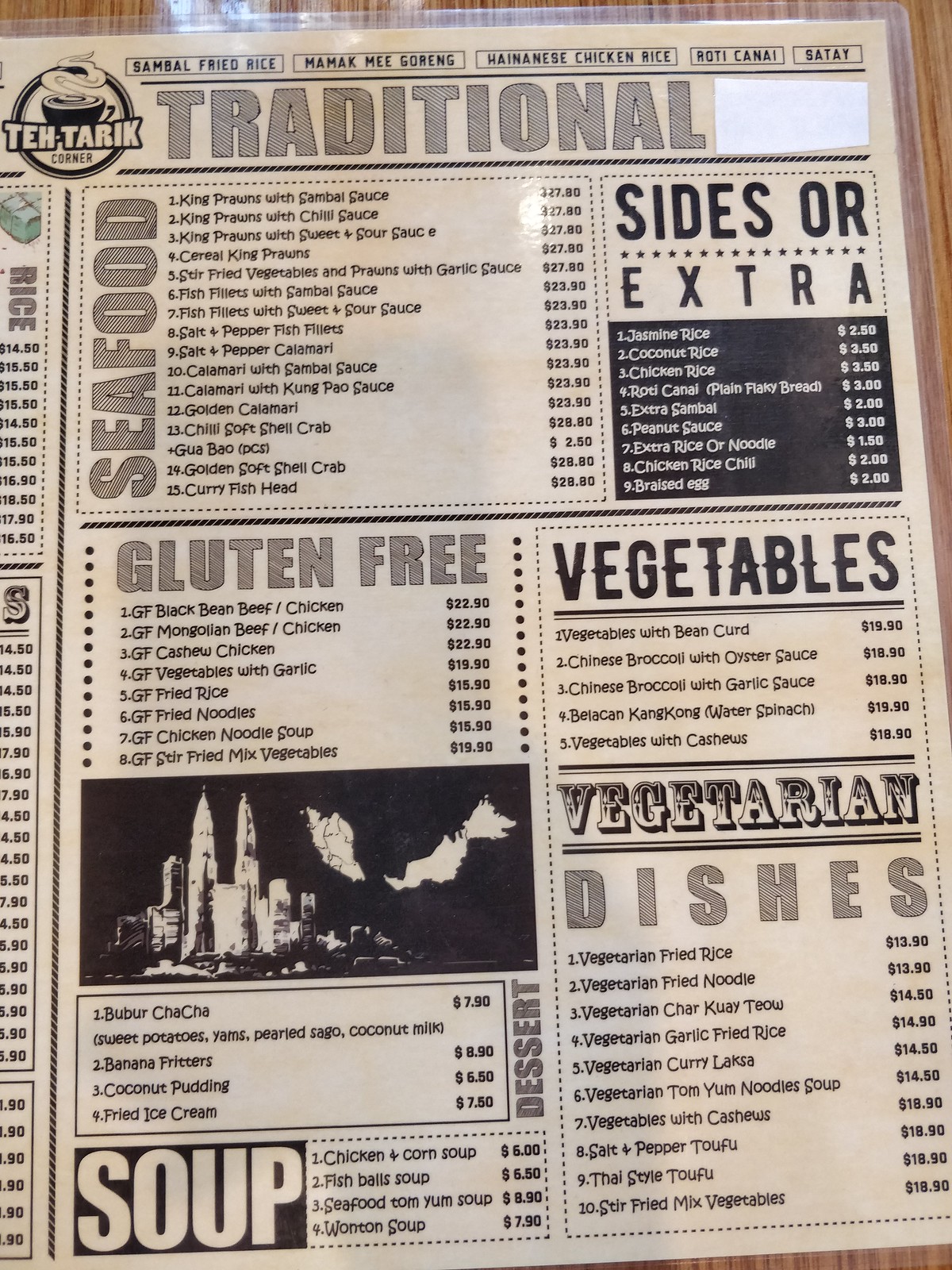The image depicts a vertically oriented menu set against a medium brown wooden table with darker streaks, giving the scene a warm, rustic feel. The menu itself has an aged, beige appearance, with black text and small black rectangular callouts organizing the information. At the top of the menu, there is a circular emblem featuring the words "Teh Tarik" and an illustration of a steaming beverage, perhaps coffee or tea. 

Prominently displayed in large, bold, gray letters is the word "Traditional," emphasizing the classic nature of the offerings. The food items are sectioned into various categories: "Seafood," which is uniquely listed sideways from the bottom up; "Sides or Extras"; "Gluten-Free"; "Vegetables"; "Vegetarian Dishes"; and "Soup." Additionally, there is a black cut-out graphic at the bottom featuring silhouettes of different buildings. Each food item is accompanied by its respective price, neatly arranged for ease of reading. Overall, the menu exudes a homely, traditional charm reflective of the restaurant's ambiance.